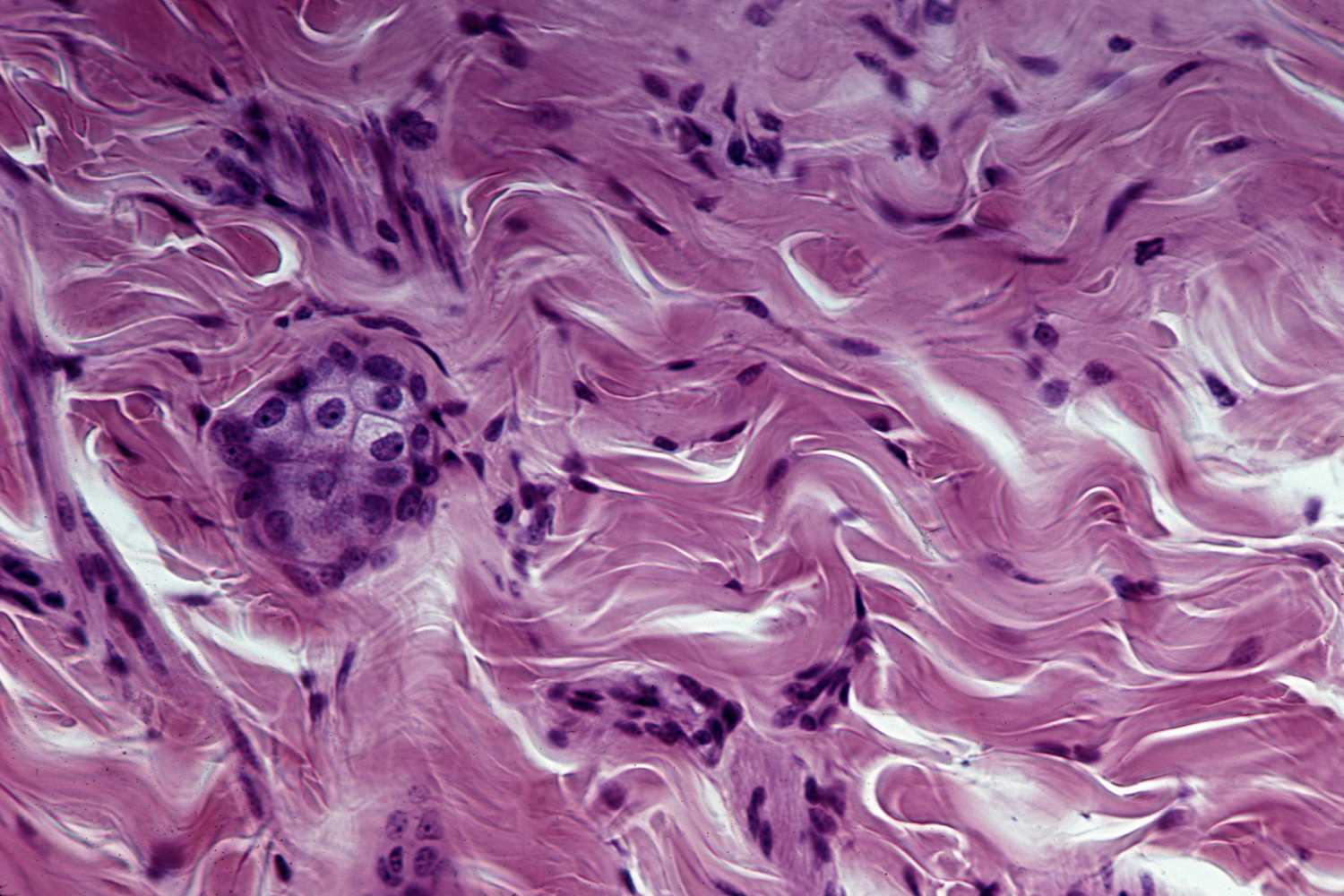A vibrant image dominated by a light purple background showcases a fascinating biological scene. On the left side of the image, a distinct cluster of irregularly shaped cells stands out, each housing dark purple nuclei. These cells resemble small rounded clumps or "raisins" clustered together, creating an organic texture against the lighter purple backdrop. Scattered throughout are numerous dark purple patches or dots, contributing to an abstract, almost painterly quality. The visual complexity is heightened by wispy white lines that weave through the background, reminiscent of wind or the fibrous strands of cotton candy. The overall composition, with its blend of maroon and violet shades and the intricate cellular details, creates a striking and somewhat surreal depiction, as if viewed under a microscope or through the lens of an artist.